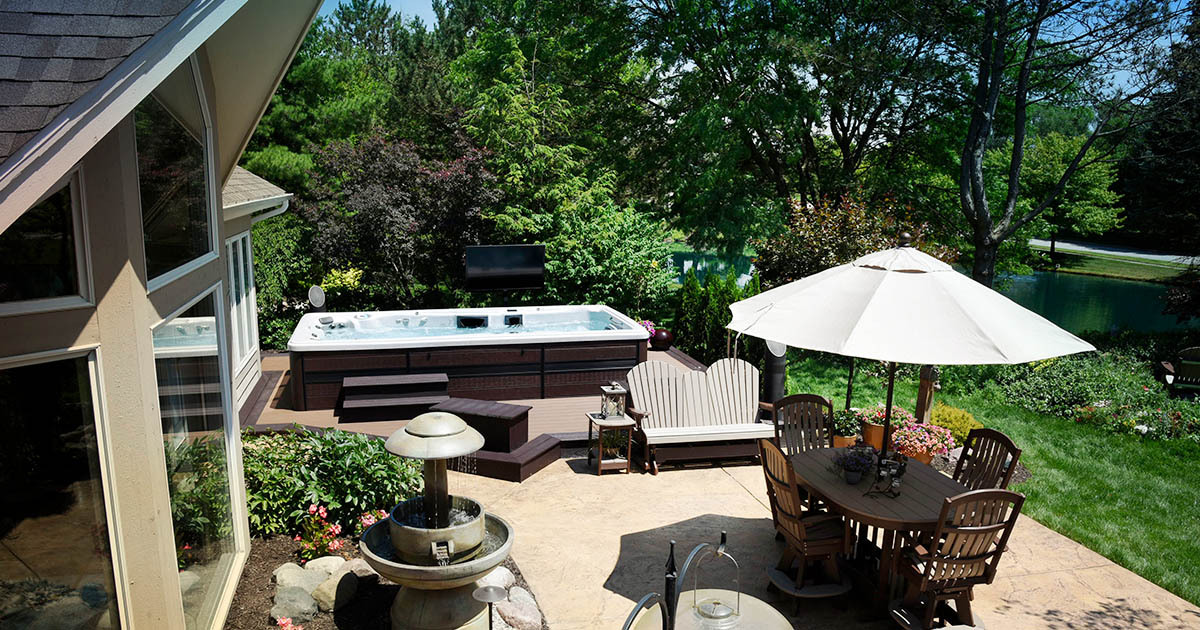This color aerial photograph captures a beautifully outfitted backyard deck of a home, bathed in daylight. At the forefront of the image, the deck itself is strikingly detailed with its intricately designed elements. Centrally located towards the back, there's a large hot tub capable of accommodating eight to ten people, complete with steps leading up to it. This luxurious feature is set against a backdrop of lush greenery, including a well-manicured lawn and garden area, and is bordered by tall, robust trees. Beyond the trees, a serene lake or possibly a pond adds to the picturesque landscape.

To the right of the hot tub, there is a wooden dinner table with four matching chairs, shaded by an umbrella poking up from its center. This setup is perfect for outdoor dining and relaxation. On the left, amid the landscaping, there's an elegant water fountain feature adding a tranquil touch. The edge of the house can be seen to the left side of the image, featuring large plate glass windows that showcase a clear view of the deck and the surrounding scenery.

Additionally, there is a charcoal grill situated behind the hot tub, and a two-person chair nearby, enhancing the deck's utility for both leisurely and functional purposes. The vegetation continues beyond the backyard, adding layers of depth with various trees, bushes, and grassy areas. Another notable element is a road barely visible on the far right, suggesting a connection to the broader environment. The entire scene is bathed in sunlight, highlighting the vibrancy and inviting nature of this idyllic backyard retreat.